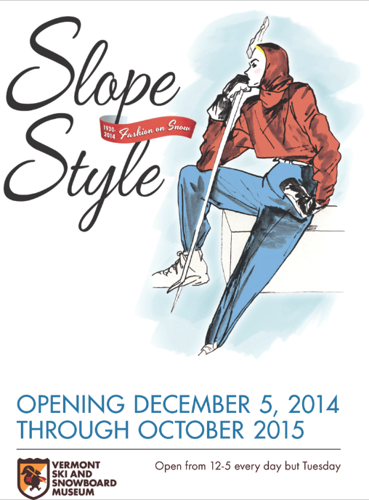The poster titled "Slope Style" is set against a white background with a black line at the top. The title "Slope Style" is written in a bold black cursive font near the top left, accompanied by a small red banner mentioning "1930 to 2014 fashion and snow." Below this, there is an illustration of a woman wearing a red top with a hood, blue pants, and white shoes, seated on a white block, holding a ski pole with a blue background behind her. The poster announces an event opening on December 5th, 2014, running through October 2015, in blue font. Beneath this, there is a shield logo with a squirrel, set against an orange and white background, associated with the Vermont Ski and Snowboard Museum. The text "Vermont Ski and Snowboard Museum" is bold and black. To the right of the logo, it states that the museum is open from 12 to 5 every day except Tuesday.